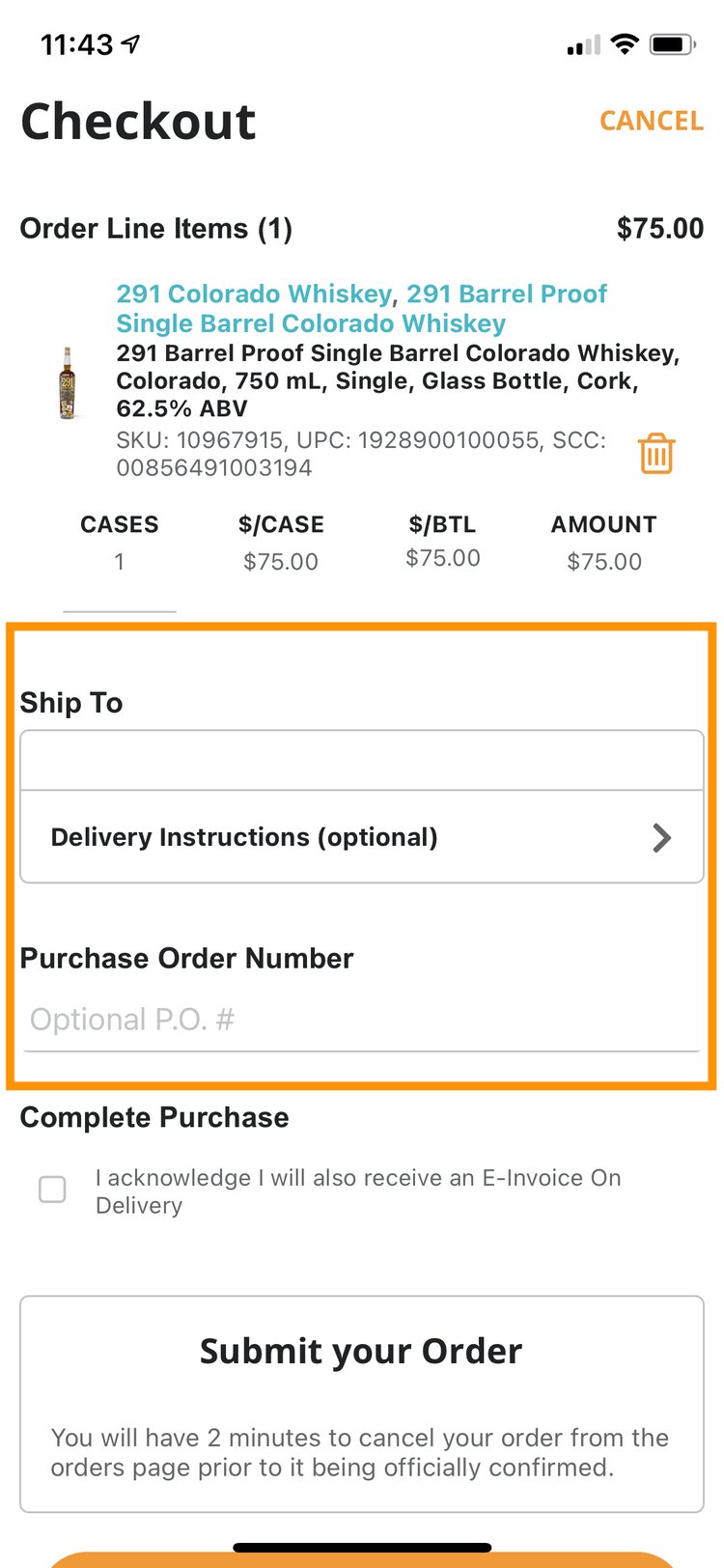This is a detailed screenshot of a mobile checkout page for purchasing liquor, specifically a 291 Colorado Whiskey. At the top left corner, the word "Checkout" is prominently displayed. On the top right corner, there's a "Cancel" option. Directly below the "Cancel" text, the total amount due is shown, which is $75.

The main focal point of the checkout page is the detailed listing of the purchase item: a 291 Colorado Whiskey, specifically described as a 291 Barrel Proof Single Barrel Colorado Whiskey. The SKU number for the item is 1096-7915, and the UPC code is 1928-9001-00055. On the left of this detailed information, there is an image of the whiskey bottle.

Additionally, there is a trash icon for removing the item from the cart, indicating the quantity is one case, along with the total item cost of $75.

Below the item description, there is a section bordered in an orange box labeled "Ship To." This section includes a field for "Delivery Instructions." There is also a place for entering a "Purchase Order Number," which is currently blank.

Further down, there's a line with the text "Complete Purchase" next to a checkbox stating, "I acknowledge I will also receive an e-invoice on delivery."

At the bottom of the page, prominently displayed, is a "Submit Your Order" button. There is a note indicating that the user has two minutes to cancel the order from the order page before it becomes officially confirmed.